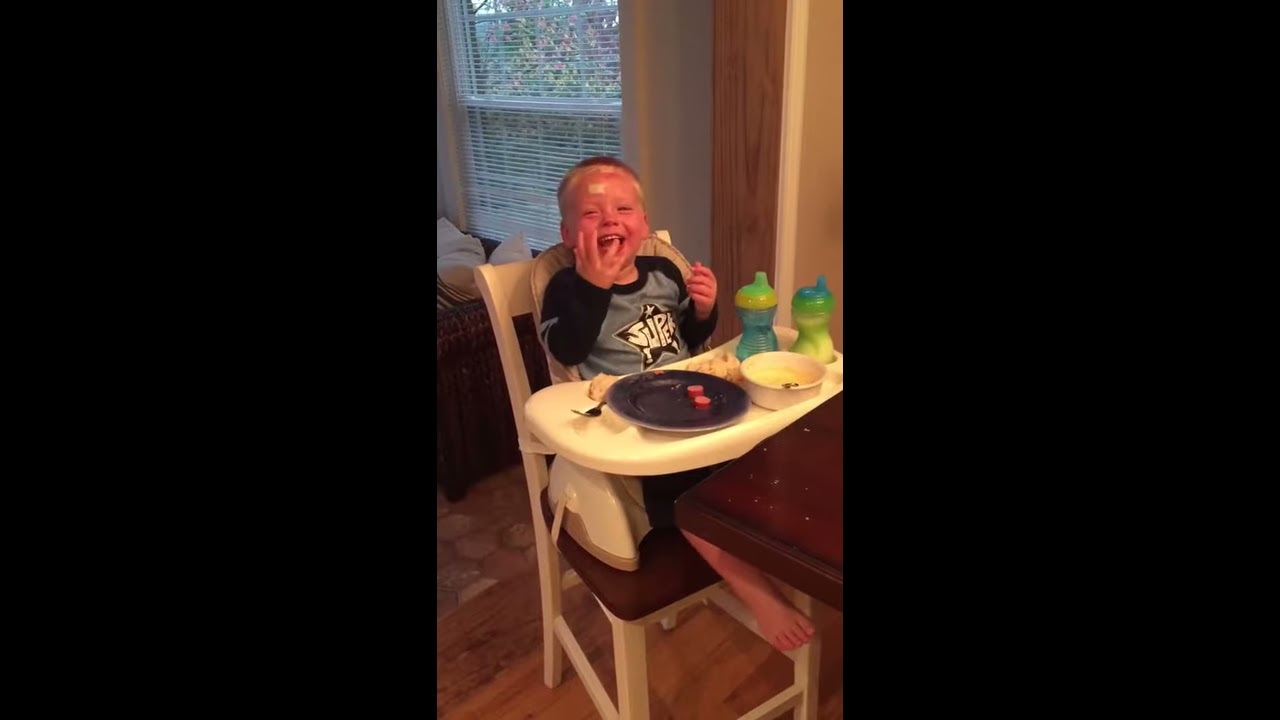In this vibrant indoor scene, a young boy is joyfully seated in a high chair, wearing a gray and black long-sleeved shirt adorned with a star that reads "Super." His laughter lights up the photograph as he looks directly at the camera, one hand raised in front of his smiling face. The boy appears to have a bandaid on his forehead, possibly from a recent bump. 

The high chair features a tray with a black plate holding cut-up pieces of hot dog, a white bowl of cereal or soup, a fork, and a spoon. Two colorful sippy cups are also on the tray—one blue with a green and yellow top, and one green with a blue and dark green top. 

The backdrop includes a window with white Venetian blinds, through which daylight pours in, vaguely illuminating an outdoor view of trees. The floor underneath is wood, adding a warm, homely touch to the setting.